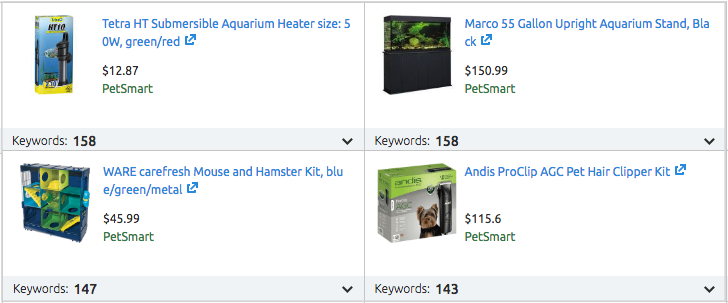The image displays a gray-outlined rectangle that is subdivided into four equal sections by a horizontal and a vertical line intersecting at the center. Each section features different product information in a combination of blue, black, and green text, corresponding to various items available at PetSmart.

1. **Top Left Section:**
   - **Product Name:** Tetra HT Submersible Aquarium Heater 
   - **Details:** Size: 5 OW, Green/Red 
   - **Price:** $12.87 (in black) 
   - **Retailer:** PetSmart (in green)
   - **Keywords:** 158 (in green)
   
2. **Bottom Left Section:**
   - **Product Name:** Weacare Fresh Mouse and Hamster Kit
   - **Details:** BLU, ESO Blue/Green/Metal
   - **Price:** $45.99 (in black) 
   - **Retailer:** PetSmart (in green)
   - **Keywords:** 147 (in green)
   
3. **Top Right Section:**
   - **Product Name:** Marco 55-Gallon Upright Aquarium Stand 
   - **Details:** Color: Black 
   - **Price:** $150.99 (in black) 
   - **Retailer:** PetSmart (in green)
   - **Keywords:** 158 (in green)
   
4. **Bottom Right Section:**
   - **Product Name:** Andis Pearl Clip AGC Pet Care Hair Clipper Kit 
   - **Price:** $115.60 (in black) 
   - **Retailer:** PetSmart (in green)
   - **Keywords:** 143 (in green)